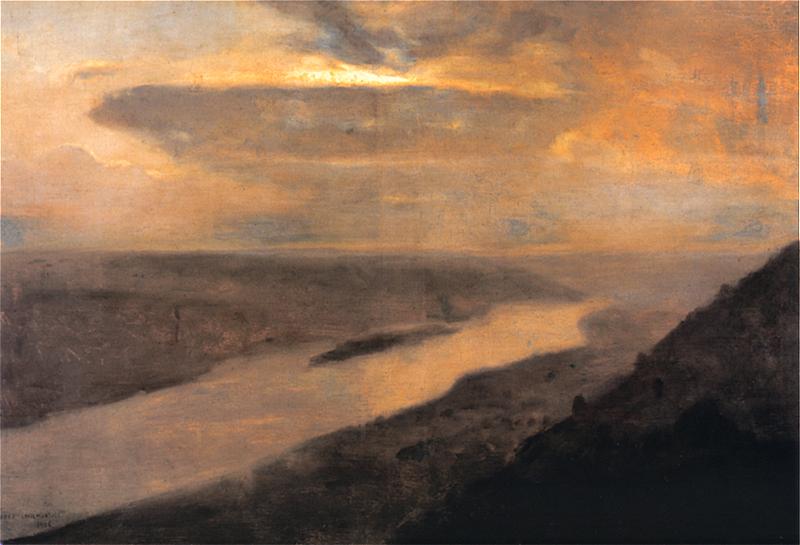This artwork captures a serene and abstract landscape at sunset, characterized by its impressionistic style. The foreground features a dark, almost black hill in the bottom right corner, which gradually transitions to lighter shades of gray as it moves upward. A stream of water begins in the lower left and meanders towards the middle of the painting, bordered by elevated land on the left and an incline leading to another hill on the right. The stream and surrounding land are rendered with shades of brown, gray, and hints of white. Overhead, the sky is an evocative blend of peach, orange, light gray, and a small patch of blue, suggesting an overcast sunset. The painting is devoid of any buildings or people, focusing solely on the natural elements. The artist's signature is subtly placed at the bottom left, though it is not clearly legible.